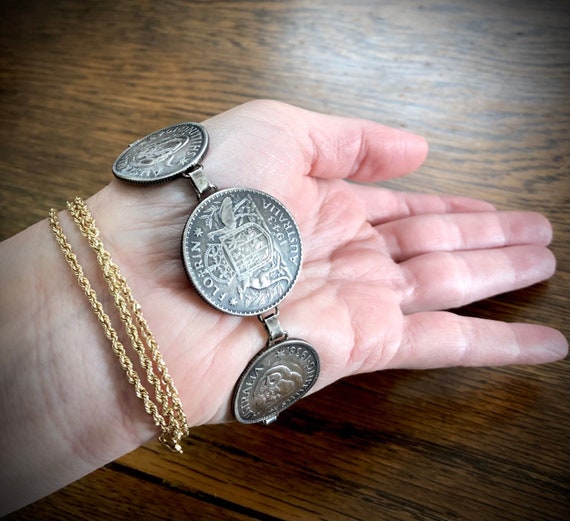This square photograph features a close-up of an elderly woman's left hand, palm up, resting on a dark woodgrain table. The hand prominently displays two distinct bracelets: one is a delicate gold chain bracelet with three links wrapped around her wrist, and the other is a more unusual piece made up of at least three old Australian coins. These coins, dark bronze in color, are intricately etched and feature the text "Florin Australia 1943," a coat of arms flanked by a kangaroo and an emu, and possibly a "Schilling" from 1938. The coins are arrayed in a way that they span from the woman's wrist to the meat of her palm, showcasing their historical details. The image captures the warmth and texture of both the aged hand and the worn, cherished items, set against the rich backdrop of the wooden table.